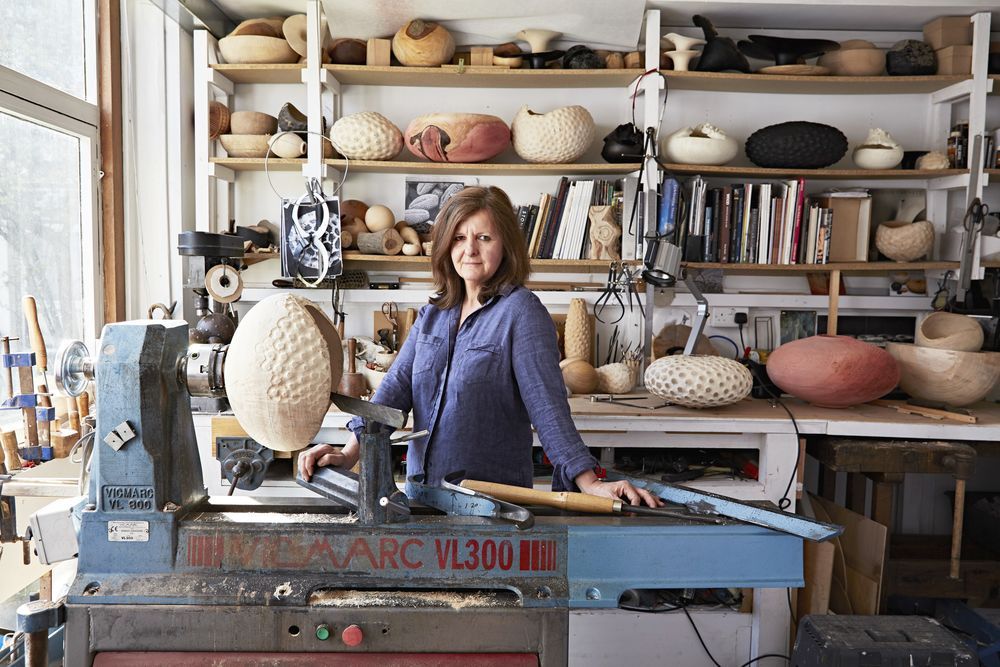A full-color, square photograph captures a bright, sunny day inside a well-lit artisan's workshop. On the far left, light pours through a large window that offers a view of trees outside. Central to the image is a middle-aged woman with shoulder-length dark hair, wearing a long-sleeved blue shirt, who is standing behind a prominent blue lathe, specifically marked as a VICMARC VL300. Mounted on the lathe is a large, roundish ceramic object, suggesting she is in the process of crafting it. Surrounding her workspace is a wooden workbench and several shelves. The shelves are populated with various round and oval-shaped ceramic bowls and vases, many resembling the object on the lathe. Books and pieces of wood also occupy some of the lower shelves, indicating a versatile artistic environment. The setup, filled with diverse materials and tools, highlights the creative atmosphere of the artisan's studio.